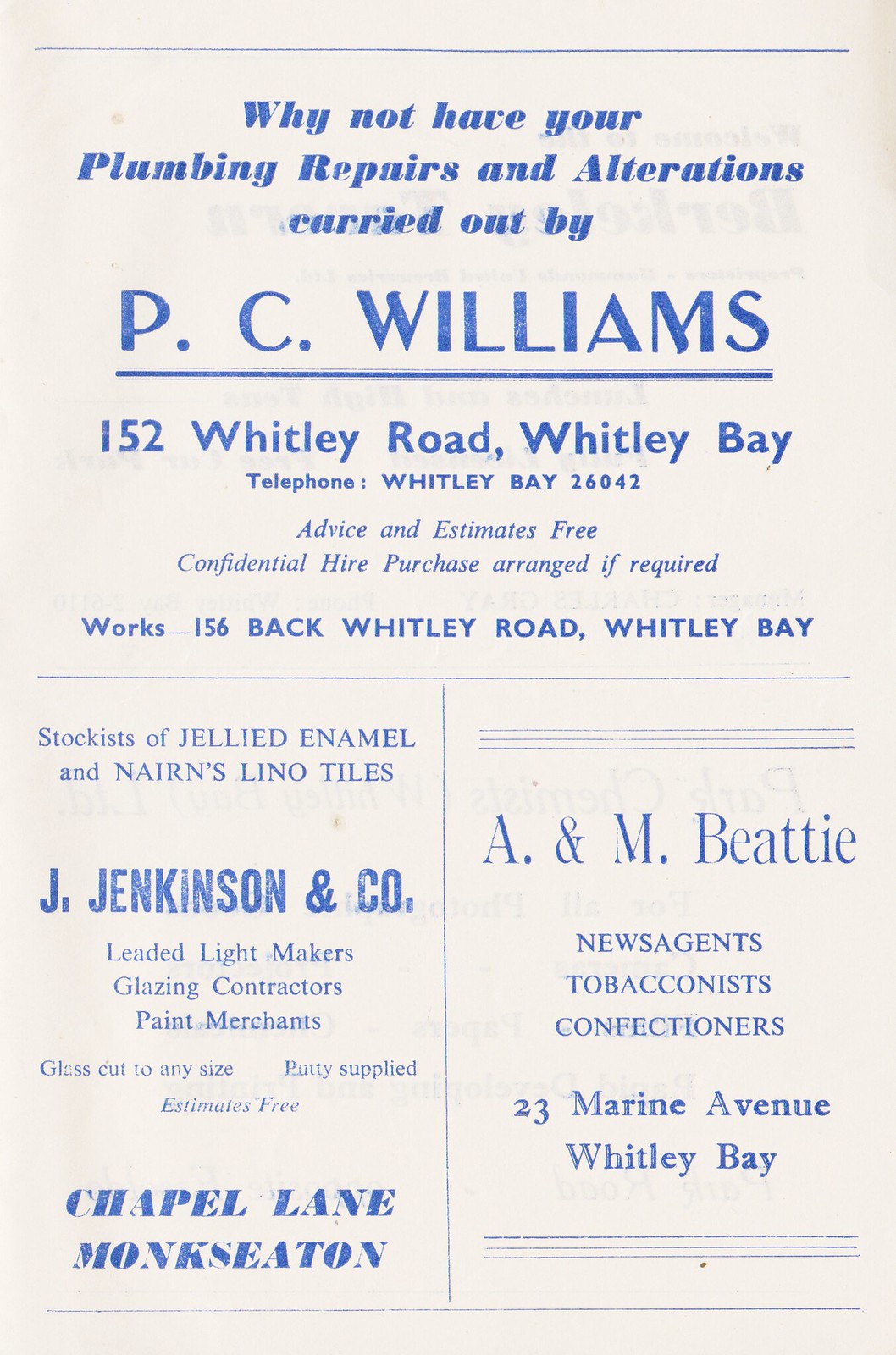The image depicts an off-white, faded piece of paper with blue printed text, likely from a program or magazine, showcasing three distinct advertisements. The top half of the page prominently features an ad for P.C. Williams. At its center, the ad encourages, "Why not have your plumbing repairs and alterations carried out by P.C. Williams," followed by their address at 152 Whitley Road, Whitley Bay, and the telephone number Whitley Bay 26042. It also offers "advice and estimates free, confidential hire purchase arranged if required," and mentions a secondary works address at 156 Back Whitley Road, Whitley Bay.

In the lower half of the page, the left section is dedicated to J. Jenkinson & Company, advertising their services as stockists of jellied enamel and Naren's lino tiles. They also highlight their expertise as leaded light makers, glazing contractors, and paint merchants, with their location specified at Chapel Lane, Monkseaton. 

The right section of the lower half contains an advertisement for A&M Beattie. This ad promotes their business as newsagents, tobacconists, and confectioners located at 23 Marine Avenue, Whitley Bay. Each advertisement is neatly formatted in blue text against a very pale blue background, creating a cohesive and visually appealing layout.